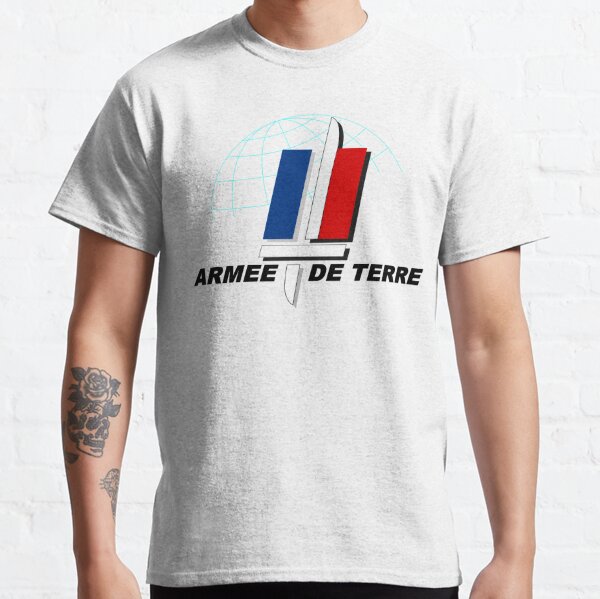The photograph depicts a Caucasian model from the hips up, with the head and legs out of frame. The individual is wearing a plain white, short-sleeved t-shirt, which features a distinctive design at the center. This design consists of a white sword that appears to be set between a blue rectangular area on the left and a red rectangular area on the right. Additionally, the text "Arm-Made to Tear" is visible in black beneath the design. On the back of the t-shirt, a barely visible light turquoise sphere, resembling the skeleton of a globe with latitude and longitude lines, can be seen.

The model's arms are down at their sides, displaying tattoos. The right arm features a large flower tattoo on the forearm and a smaller tattoo closer to the wrist. There is also the mention of a skull tattoo, further characterizing this arm. Meanwhile, the left arm has the hint of another tattoo partially visible under the sleeve. The setting of the photograph is against a plain white background.